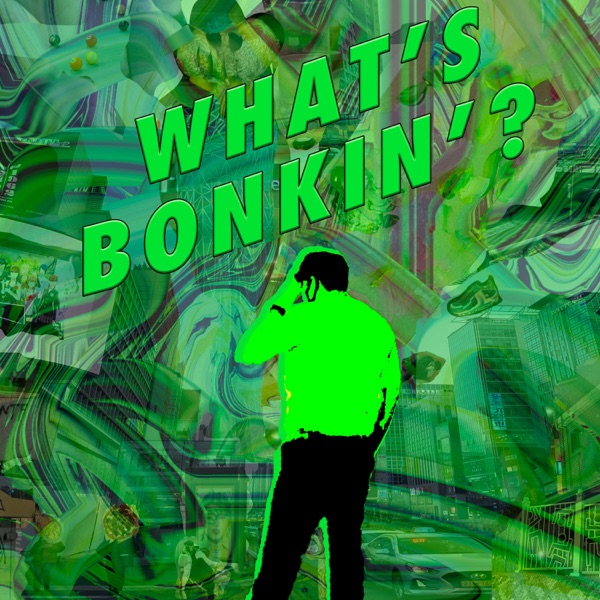The image predominantly features a collage-style background with various shades of green, swirling patterns, and a mix of other colors like purple, blue, yellow, orange, and white. In the foreground, a cartoonish figure of a man is depicted with his back to the viewer, wearing a green shirt and black pants. He appears to be holding his head with his left hand while his right hand is in his pocket. The composition is busy and vibrant, with elements of a cityscape, including buildings, Chinese letters, cars, and floating images of sneakers. There is a poster-like element on the left side featuring people in a party hat or witch's costume meshed into the green background. Prominently, the text "What's Bonkin?" in large, green capital letters ascends diagonally across the top of the image, adding a quirky and intriguing caption to the overall scene.